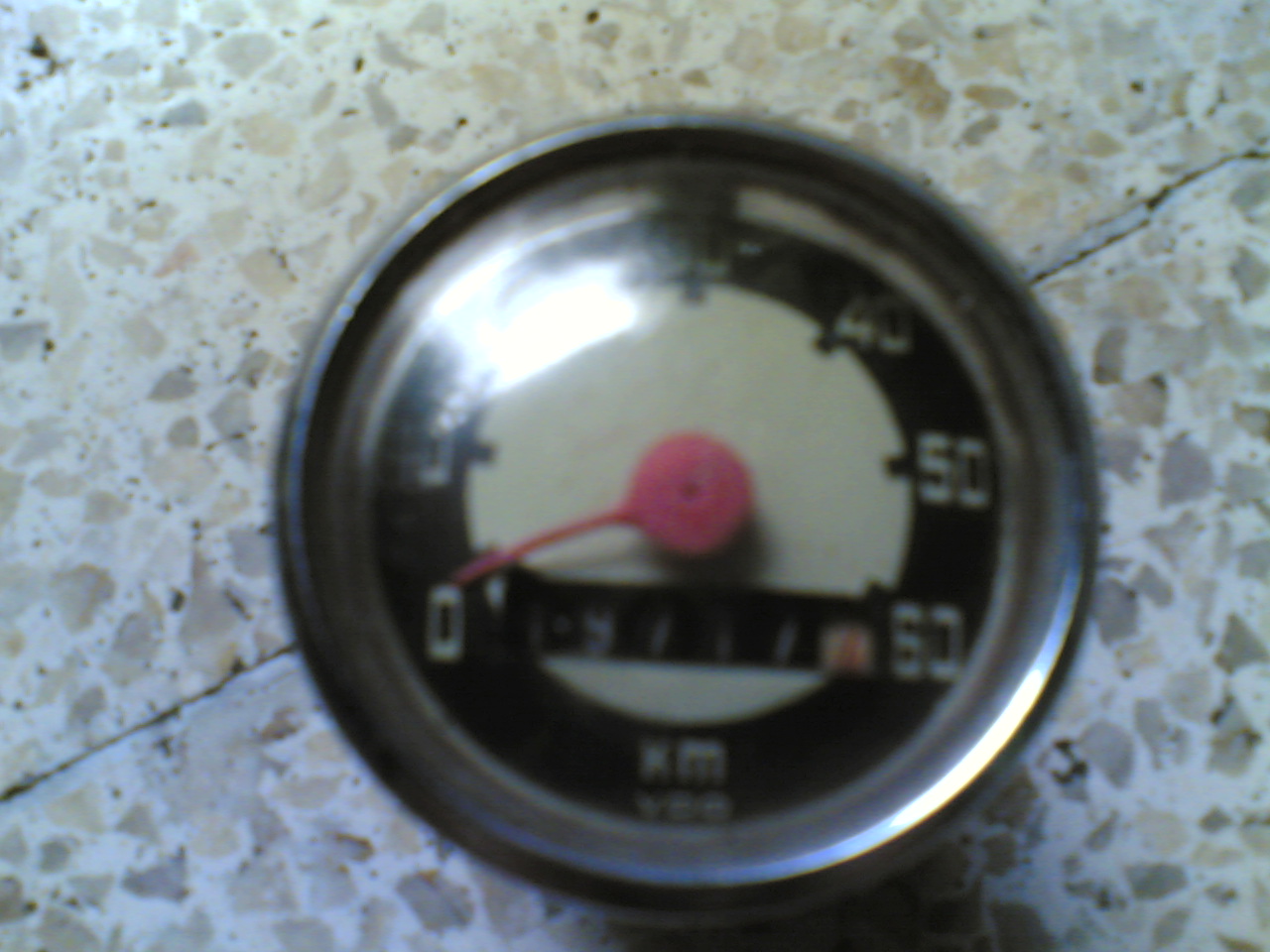This is an extremely blurry photograph depicting a metal-encased dial, likely a speedometer. The dial features numerals arranged in increments, starting from 0 at the bottom to an indistinct number, possibly 30, at the top. There are further increments marked around 40, 50, and 60, all in a white font, blending together within the metal ring. At the center of the dial is a red needle, which points towards 0. Additionally, there is a partially visible odometer displaying a reading starting with "97," though the remaining digits are unclear. The entire device, likely from a car, bicycle, or motorcycle, rests on a brown and white terracotta surface that features a prominent diagonal crack running from the bottom left to the top right corner.